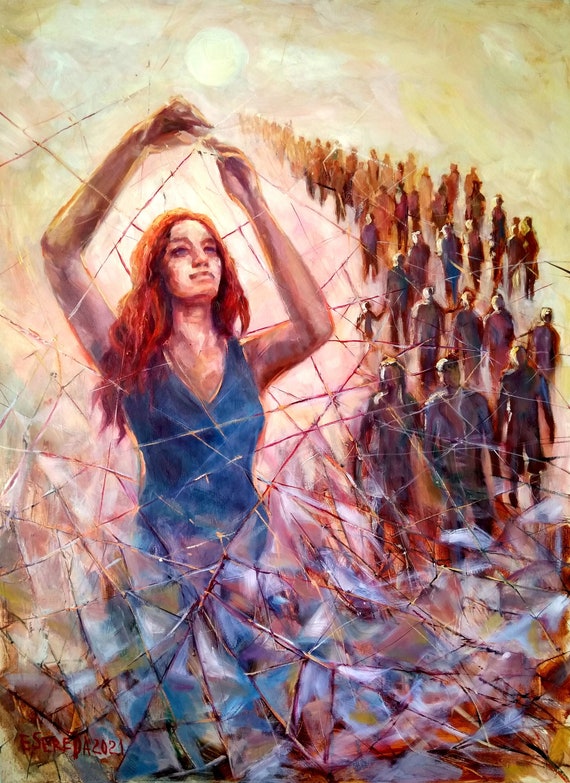This image portrays a striking painting of a woman with long red hair cascading down to her chest, wearing a sleeveless blue dress with a low v-neck. She stands with her hands raised, possibly sewing or holding something above her head. The background is a textured mix of yellow and white, and the lower portion of the painting features a cracked, ice-like design giving the impression of fractured glass. Surrounding the woman are artistic renditions of people—silhouetted figures without facial details, arranged in a long, almost endless line that stretches into the distance. These figures, painted in varying hues of violet and red, include children holding hands with adults, evoking a sense of movement and direction, as if they are following the woman. There is also an artist's signature or text in red at the bottom left, with part of the date "2021" visible. The overall composition exudes a sense of unity and guidance, with the woman seemingly leading the faceless crowd.